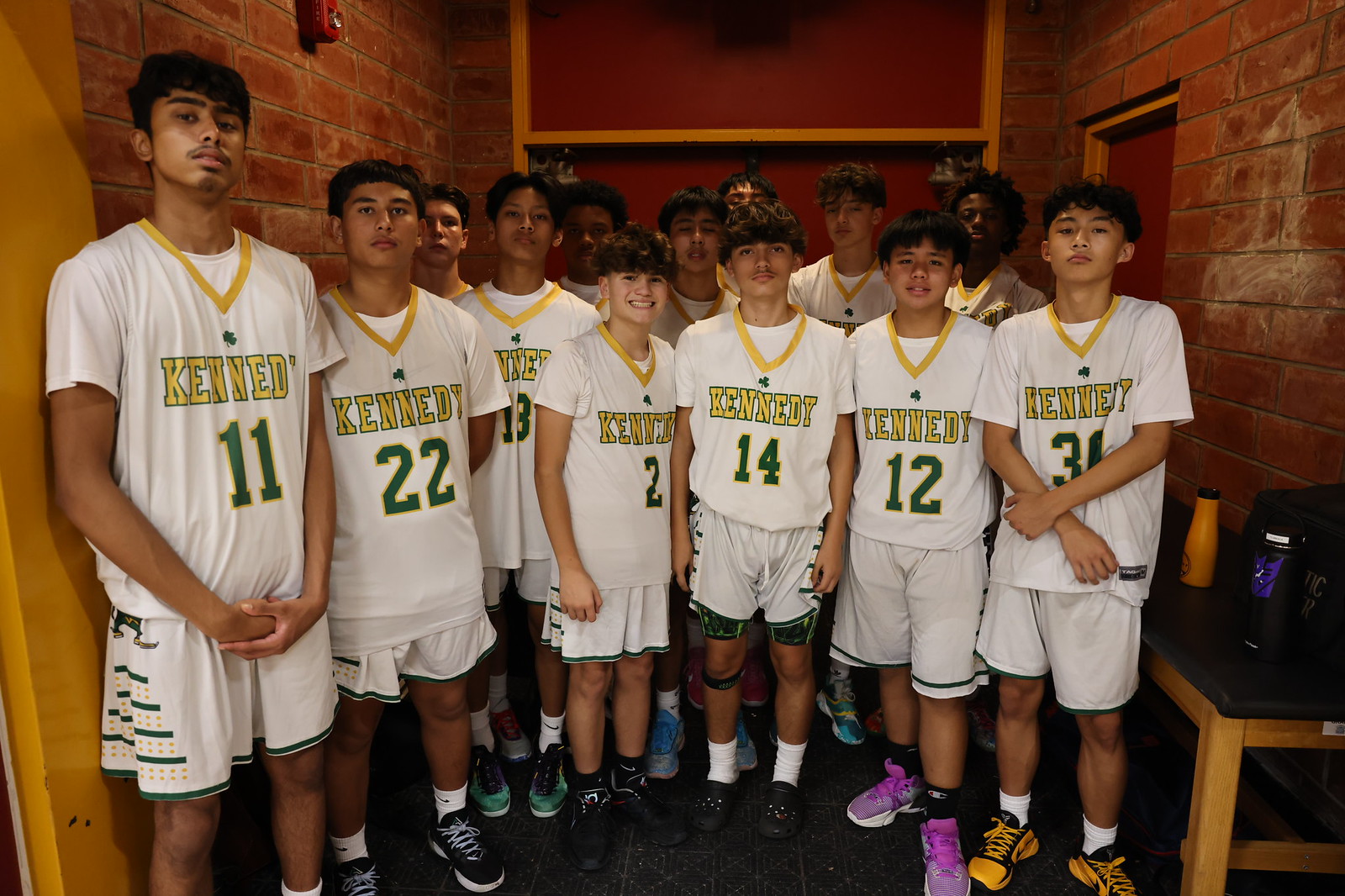The photograph depicts a group of thirteen boys from a sports team, likely soccer or football, all wearing matching white uniforms with green numbers and the name "Kennedy" written in yellow letters outlined in green. Above the word "Kennedy," there is a green three-leaf clover. The uniforms consist of white shirts with v-neck collars that have a yellow fringe, and white shorts. The boys are standing in front of a brick wall, posing and smiling, except for one in the number 14 jersey, who is looking straight at the camera with a serious expression. They are in a small room, and there is a table visible to the right of them.